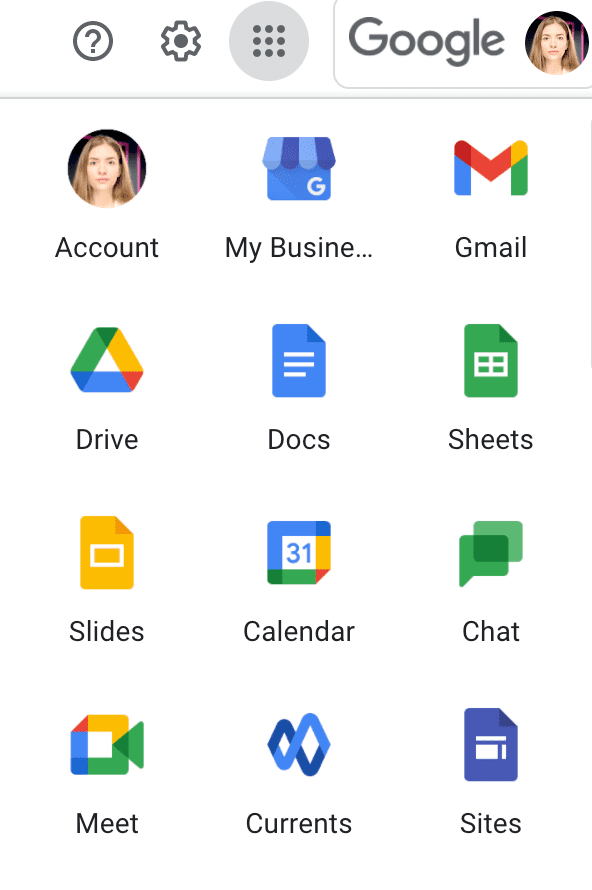The screenshot appears to be taken on a phone, showcasing various apps against a white background. At the very top, there is a toolbar featuring a circle with a question mark, a gear icon for settings, and a grid of nine dots arranged in a three-by-three formation inside a grayish circle, representing the menu. The word "Google" is prominently displayed next to a profile picture of a girl with blonde hair.

Below this toolbar, there are four rows of app icons, each labeled with their respective names:

1. **First Row:**
   - **Accounts**: Represented by a circle with a profile picture.
   - **My Business**: Depicted as a small shop icon with a "G" at the bottom right.
   - **Gmail**: Icon of a colorful "M".
   - **Drive**: Icon of a colorful triangle.

2. **Second Row:**
   - **Docs**: Represented by a blue document with white lines.
   - **Sheets**: A green icon with a chart.
   - **Slides**: A yellow icon with a rectangular shape.
   - **Calendar**: A multicolored calendar icon.

3. **Third Row:**
   - **Chat**: Featuring two green conversation bubbles.
   - **Meet**: An icon with various colors.
   - **Currents**: A blue icon resembling a sideways infinity symbol.
   - **Sites**: A blue rectangle with a white emblem.

The layout is organized and visually inviting, providing easy access to frequently used Google services and other business-related apps.